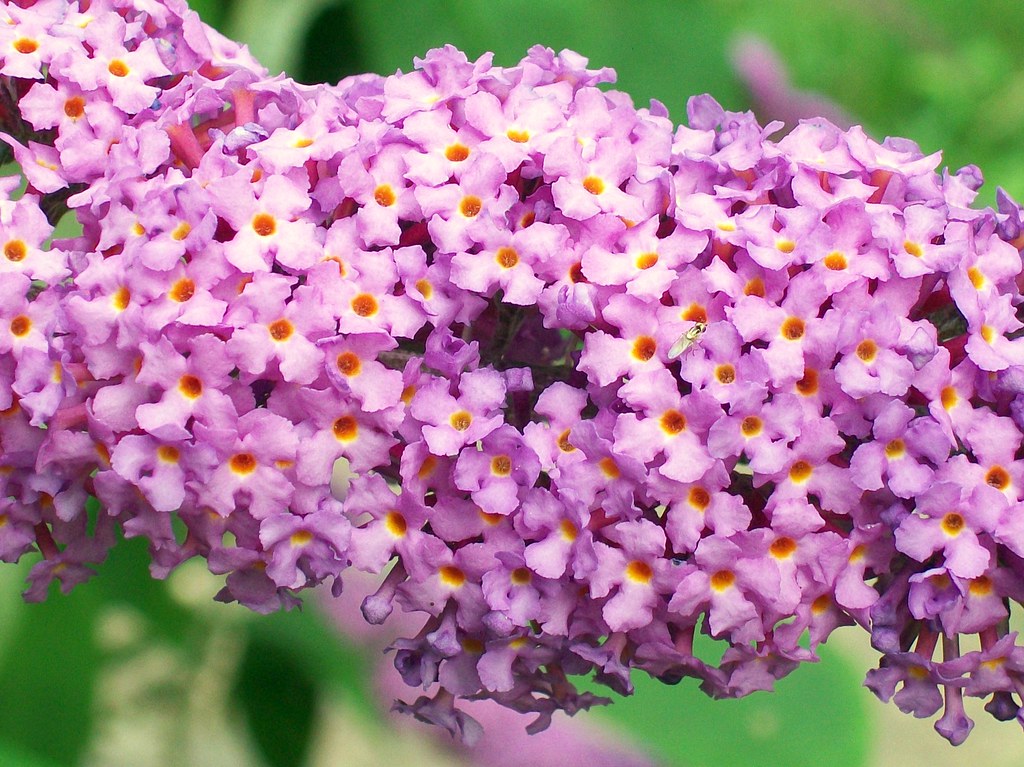This image showcases a dense cluster of small, vibrant purple flowers, each adorned with a distinct orange center encircled by a delicate white ring. The flowers appear to be tightly grouped on a branch, although the branch itself is difficult to discern. Peering into the clusters, a subtle darkness within the flowers is noticeable. A small green and yellow insect is perched at the center of this floral assembly. The blurred background hints at a natural setting, featuring assorted vegetation including grass and leaves. Additional purple elements are present in the background, though they are not clearly defined.